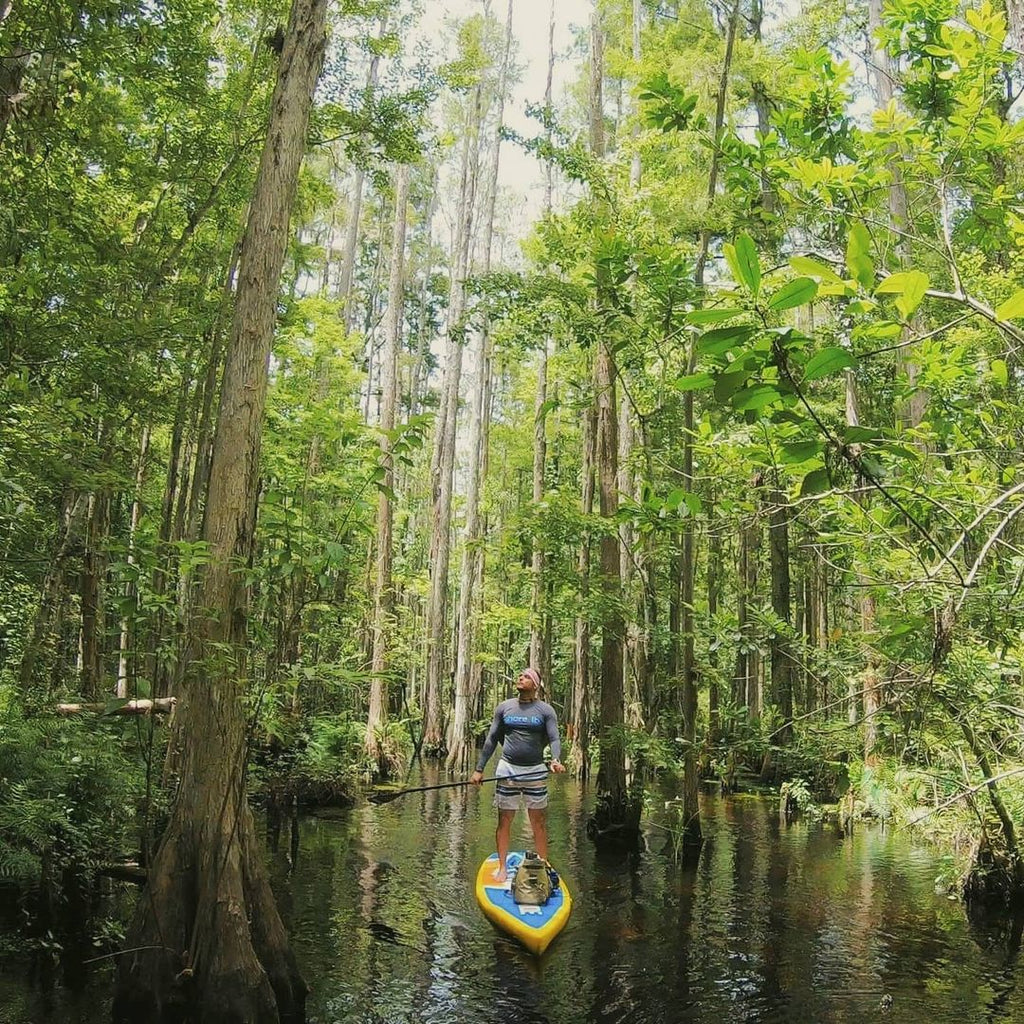In this outdoor, daytime image, a man is captured standing upright on a small yellow kayak with blue accents, holding a paddle in his hand. He's looking upwards and to the left, suggesting he might be taking in the surroundings or observing something above. The man is dressed in a long-sleeved, dark-colored shirt featuring blue print, although the exact details of the print are unclear, and he's paired it with off-white shorts adorned with yellow and darker stripes. He appears to be wearing a headband or possibly a hat and has a small backpack placed in front of him on the kayak. The water beneath him is calm, dark, and lightly rippled, set against a backdrop of a densely forested area with tall, lush green trees stretching high into the sky. Despite the thick canopy, patches of daylight filter through, indicating a cloudy yet warm day in this serene, wooded locale.